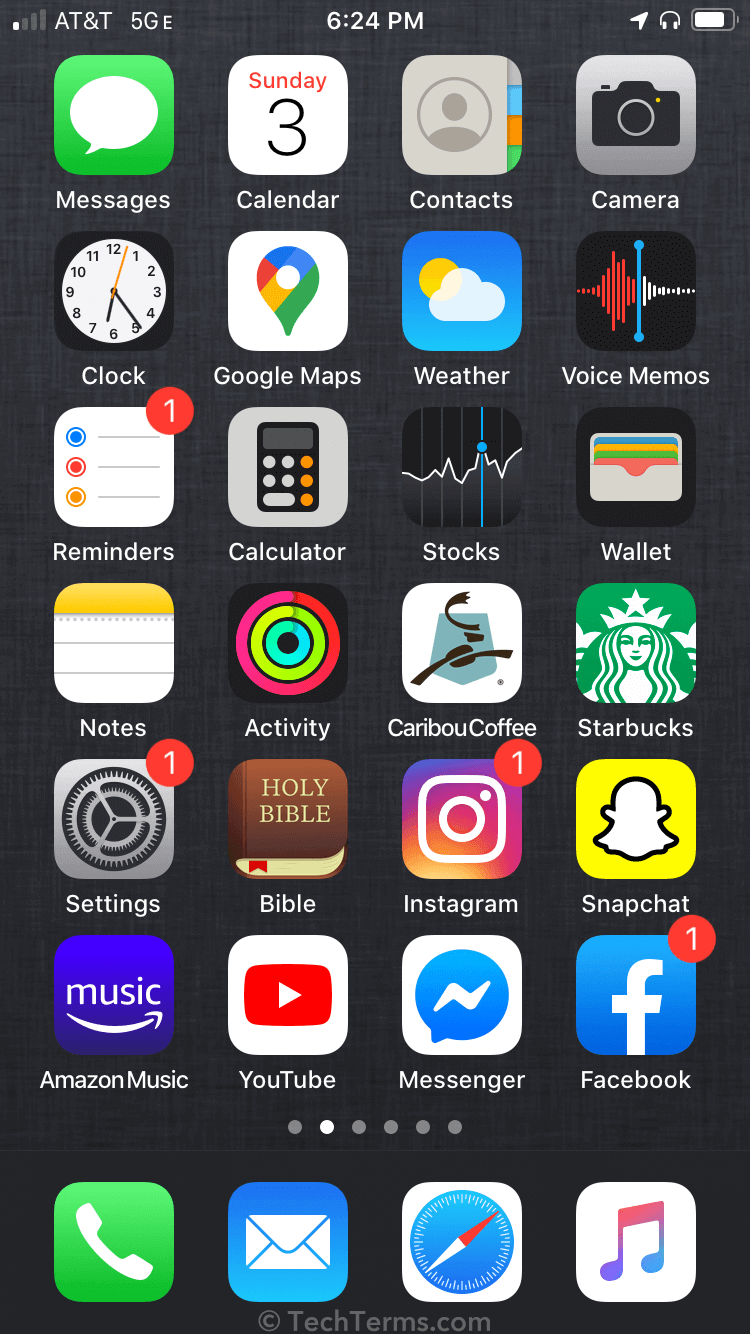This is a detailed screenshot of an iPhone's home screen, currently displaying the second page of apps as indicated by the six dots at the bottom, with the second dot highlighted. The screen exhibits a total of 28 app icons arranged in a grid of seven rows, each consisting of four icons.

The background is set to black, suggesting that the phone is in night mode. At the very top of the screen, several status indicators are visible. On the left, the signal strength is displayed, followed by the carrier name "AT&T" and a "5G" icon. The center of the status bar shows the time as "6:24 PM." On the far right, there are three more icons: a location services icon, a headphones icon indicating connected audio devices, and a battery icon showing the current battery percentage.

The icons start with "Messages" located in the top-left corner of the grid. At the very bottom center of the screenshot, a watermark reads "© techterms.com," signifying the source of the image.